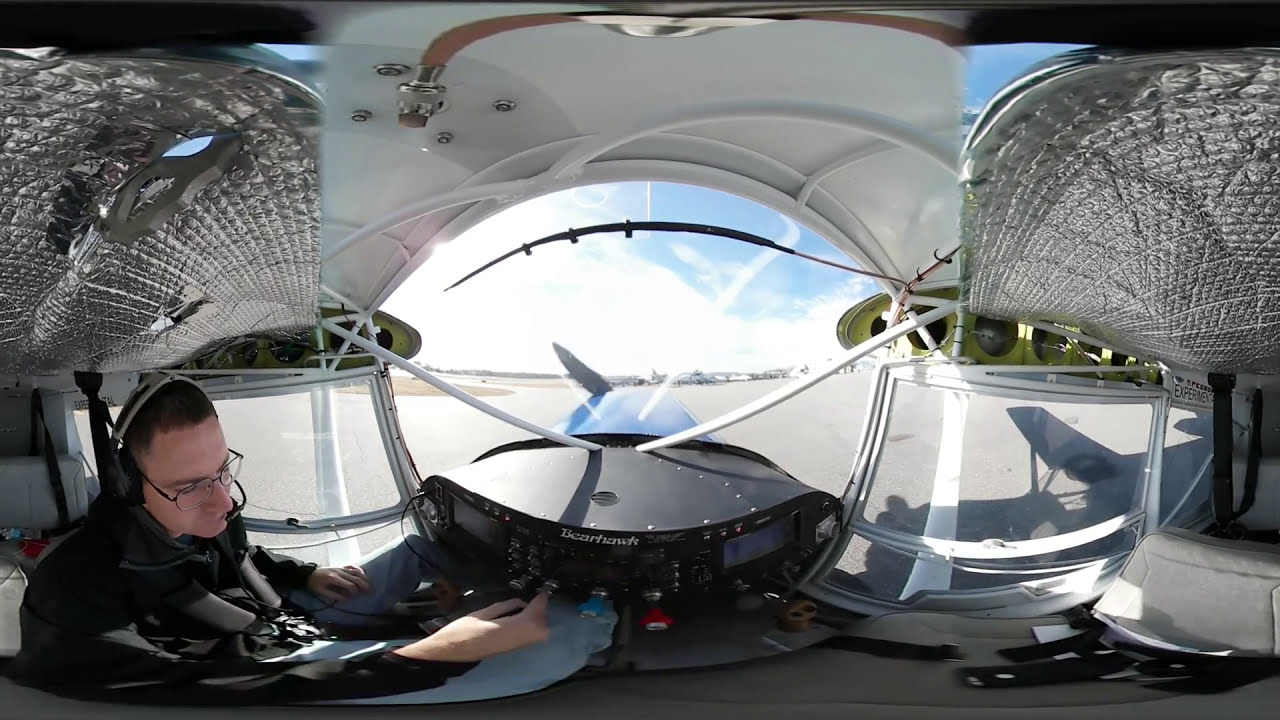A wide panoramic photograph taken from inside the control center, or cockpit, of an airplane features a detailed and immersive view of the aircraft's interior and some of its exterior components. In the top middle part of the photo, the white metal interior resembles the inside of a plane, and just below it is a distinct circular window. Through this window, you can see the narrowing blue metallic nose of the aircraft extending over a vast gray concrete runway. 

Beneath the window is a black, curved control pad equipped with several silver knobs, a big blue button, and a big red button. On the left side of the image, a man with short hair, wearing spectacles and a thick black jacket, adjusts the controls. He also has headphones on with a microphone angled towards his mouth, and appears to be looking down at a piece of paper in his hands. 

The distortion from the fish-eye lens used for the photograph makes the center of the image appear closer while the sides seem farther away. Visible through the front windshield of the airplane are the blue hood and a gray metallic propeller, accompanied by a curved windshield wiper at the top. The ceiling of the cockpit has shiny, quilted silver insulation, and an insulated yellow hose is seen at the top. The right side of the image shows additional details like another door, bells, hooks, and lighting fixtures dangling. The aircraft's shadow falls on the clear runway, indicating the photo was taken during the daytime under a clear sky while the plane is still on the ground.